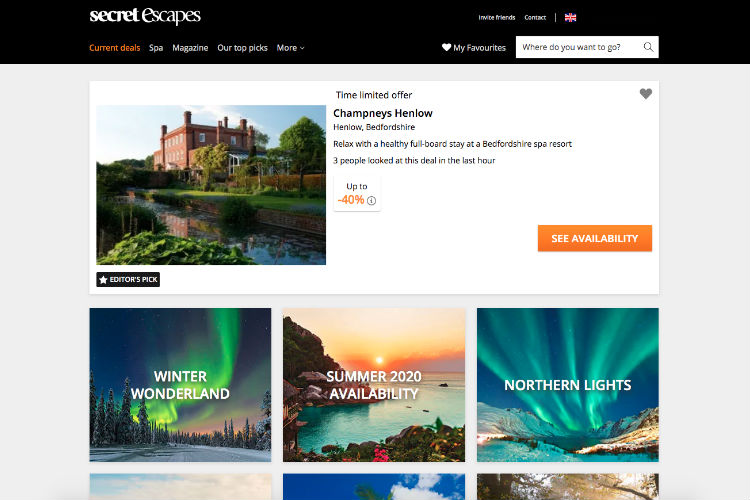The image showcases a sleek and user-friendly website layout for Secret Escapes, a travel deal platform. At the top of the page, there's a navigational menu featuring options such as Current Deals, Spa, Magazine, Our Top Picks, and a dropdown menu labeled More. Additional functionalities include inviting friends, contacting support, and changing the displayed country. 

The site also features a heart icon for 'My Favorites,' allowing users to save desirable deals, alongside a prominent search bar prompting, "Where do you want to go?"

Highlighting the page is an "Editor's Pick" section and a time-limited offer for a "Japanese Henlo in Henlo Bedford Shire," promoting a relaxing, healthy full-board stay at the Bedforshire Spa Resort with an enticing discount of up to 40%. It's noted that three people viewed this deal in the past hour. An inviting orange "See Availability" button directs users to check dates and further details.

Below this featured deal, additional travel offers are showcased, including "Winter Wonderland," "Summer 2020 Availability," and "Northern Lights," providing a range of enticing options for various travel interests.